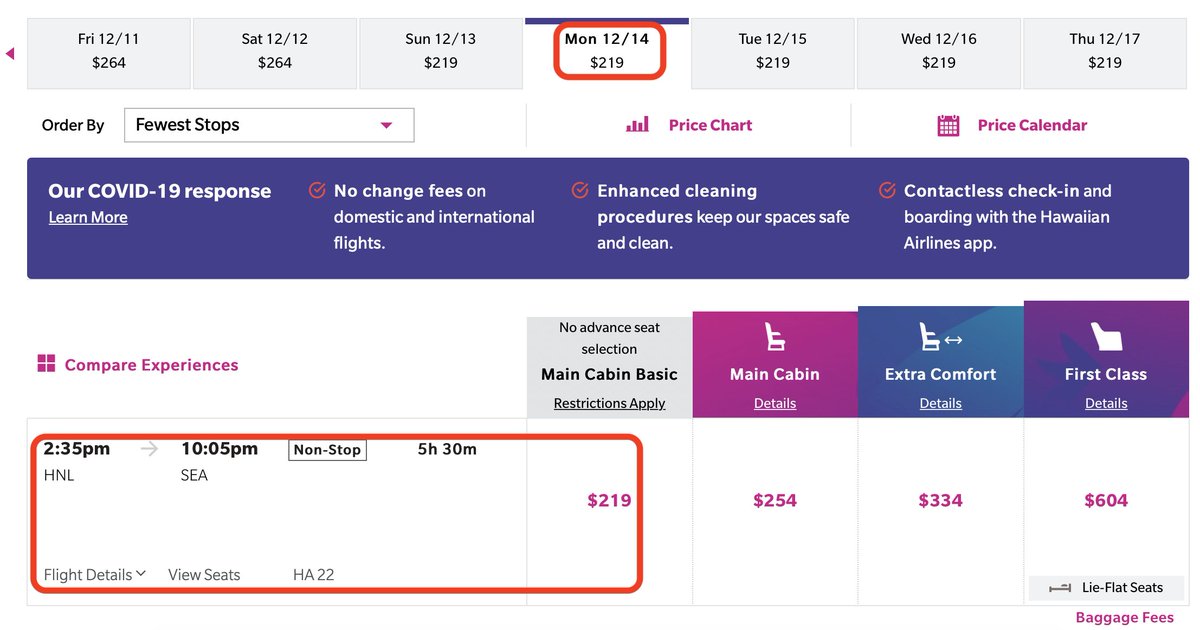A detailed screenshot of an airline website, likely Hawaiian Airlines, showcasing various booking options and information. At the top of the page, a menu allows users to select booking dates and view associated costs. The currently selected date is Monday, December 14th, with a flight priced at $219 USD. Directly below, there's a dropdown menu for selecting stops, adjacent to options for loading a price chart and performing a price calculation based on chosen stops.

A prominent purple bar below this section features a COVID response link for more information, alongside notices about no change fees for domestic and international flights, enhanced cleaning procedures, and the availability of the Hawaiian Airlines app for contactless check-in and boarding. 

The booking options are divided into clearly marked categories: Main Cabin Basic (with restrictions), Main Cabin, Extra Comfort, and First Class. These options are color-coded, with Main Cabin Basic in purple, Extra Comfort in blue, and First Class in dark purple, all featuring white text.

Further down, detailed flight information is provided: a nonstop flight departing at 2:35 PM and arriving at 10:05 PM, with a total duration of 5 hours and 30 minutes. The Main Cabin Basic fare is noted as $219 USD, while upgrade options are listed as $254 USD for Main Cabin, $334 USD for Extra Comfort, and $604 USD for First Class. Additional baggage fees are mentioned for luggage exceeding the standard allowance.

This detailed screenshot illustrates the available booking options and flight details for a user planning a trip with Hawaiian Airlines.